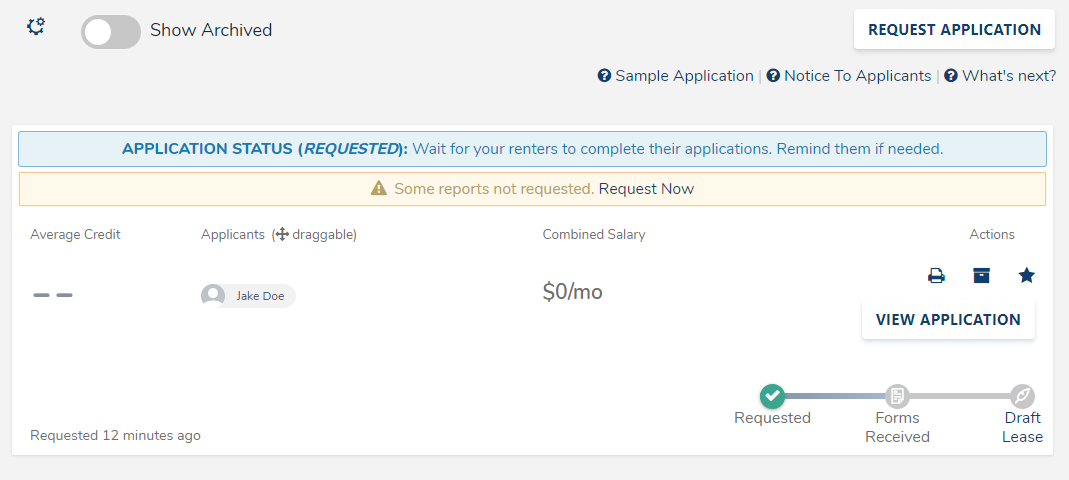In the top left corner of the image, a gear icon is situated next to a gray oval labeled "Show Archive." Following that, there is an option labeled "Request Application," then "Sample Application." Beside a question mark symbol, it states, "No just applicants, what's next?"

Below this, a blue rectangle is prominently displayed, reading “Application Status” with the status noted as "Requested." There is an instruction: "Wait for your renters to complete their applications; remind them if needed." Adjacent to this, a yellow box indicates, "Some reports not requested," with options to "Request" or "Not Request." Additional details show "Average Credit" and "Applicant Information."

Within the applicant details, there is an entry for "Jake Doe" with a combined salary of "$0 per month." Several action icons are displayed next to his name, including a printer symbol, a checkbox, and a star. The notification indicates that the application was requested 12 minutes ago. Status updates include "Forms received," and "Draft Lease."

Overall, the screen captures various stages of the rental application process, highlighting options for user actions, application statuses, and important reminders regarding the completion and submission of necessary forms.